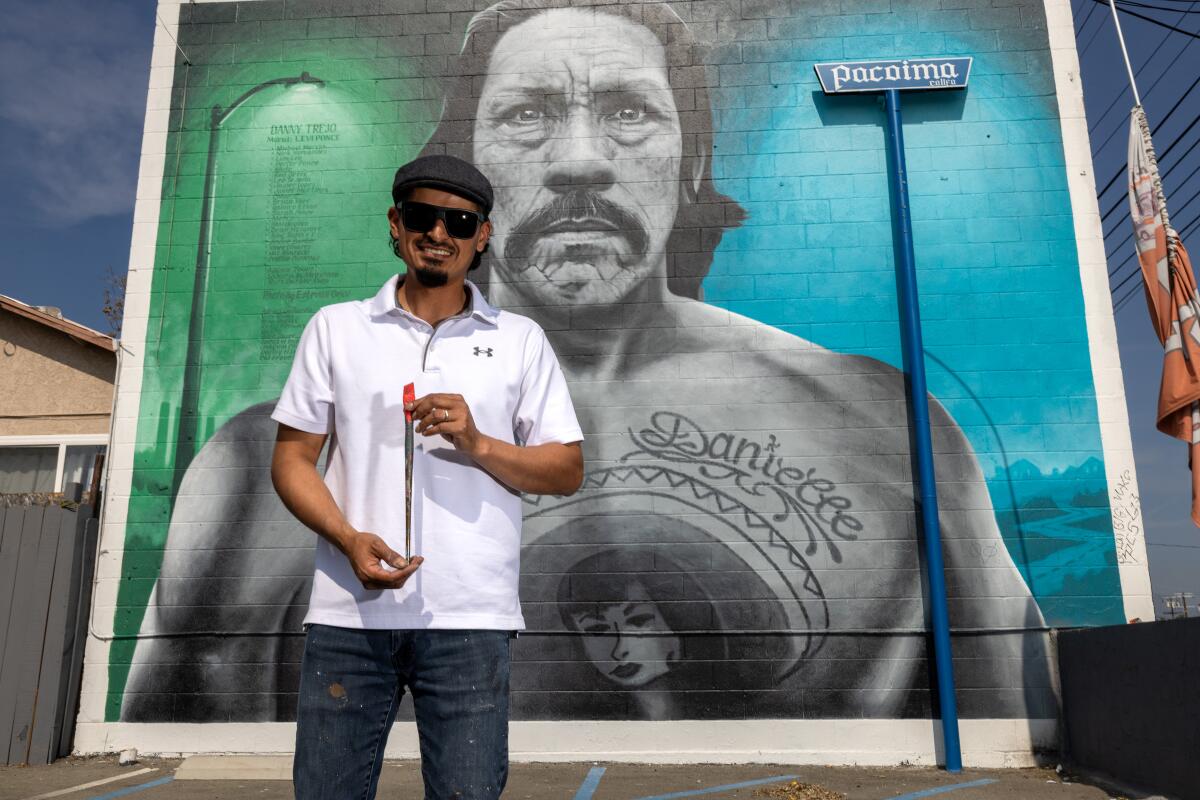A photograph captures an artist standing proudly in front of his mural painted on the brick exterior of a building. The artist, grinning broadly, is adorned with black sunglasses and a dark cap, complemented by a white short-sleeved polo shirt and paint-splattered dark denim jeans. Holding a paintbrush in his hands, he identifies himself as the creator of the striking mural behind him.

The mural itself is a grayscale rendering of Danny Trejo, featuring detailed facial hair and tattooed arms. The backdrop of the mural is split into teal and green sections, casting a striking contrast against Trejo's monochrome portrait. Next to the mural, a sign reads “PACOIMA.” The word "Danielle" is seen tattooed on Trejo's chest, which also features a black-haired woman wearing a sombrero.

In the vicinity of the mural, a multitude of objects are scattered, contributing to the bustling ambiance of the scene. A house and a table are noticeable near the wall, alongside a folded flag and an umbrella. A dumpster sits to the right, further emphasizing the urban setting of the mural. The artist's wedding ring gleams on his finger, underscoring his personal connection to the artwork he's proudly presenting.